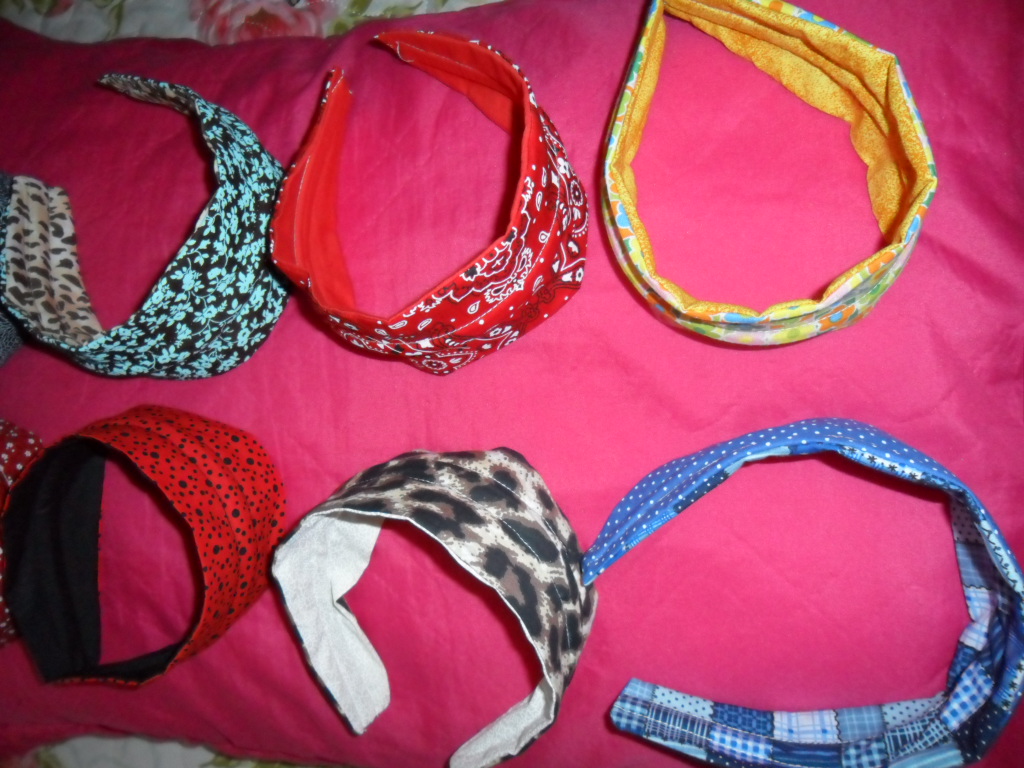The image displays six fitted head bandanas, each uniquely colored and patterned, arranged in two rows on a pink fabric background. The pink fabric, which could be a quilt or pillow, is draped over a bed with a floral comforter featuring shades of pink, blue, and white. The bandanas, appearing to have a fastening mechanism rather than traditional ties, include the following:

1. Top left: Black with white floral patterns.
2. Next to it: Red with white and black stripes and shapes.
3. Towards the right: Yellow with blue details.
4. Further right: Red with black spots.
5. Next: Gray and black camouflage.
6. Bottom right: Blue with white dots.

Each bandana is distinct in design, incorporating elements like flowers, polka dots, paisley patterns, and splotches of color, and some appear to be made from quilt-like materials.